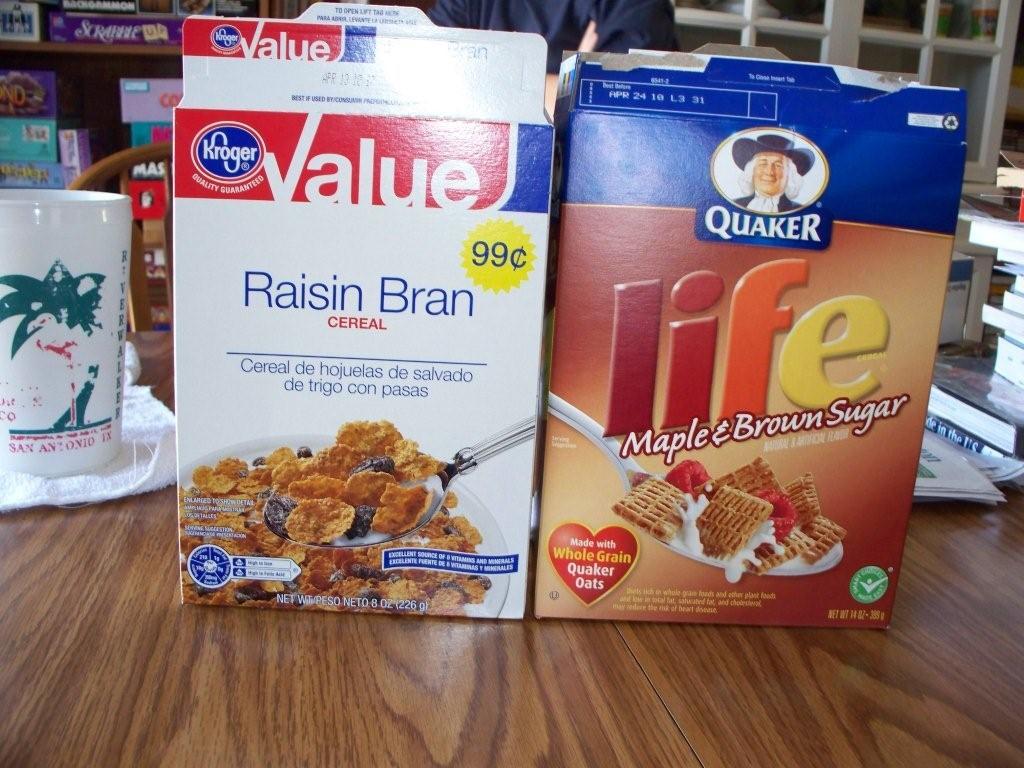The image displays a medium brown wooden table, on which the primary focus is two boxes of breakfast cereal. On the left, there is a grocery store brand box of Raisin Bran cereal from Kroger. The box is off-white with a red and blue banner at the top, featuring the Kroger logo. It prominently displays "99 cents" on a yellow sun design and includes an image of a spoon filled with Raisin Bran cereal, milk, and raisins. To the right, there is a Quaker Life cereal box with a blue upper half and a brown lower half. The box features the Quaker logo and the text "Life" in a gradient of brown, red, orange, and yellow, alongside "Maple and Brown Sugar" in white. An image of a spoon filled with Life cereal, milk, and raspberries is also visible. To the left of the Raisin Bran box is a white cup with green decorations, and behind it is a shelf containing board games, including Scrabble. Adjacent to the Life cereal box on the right is a stack of books.